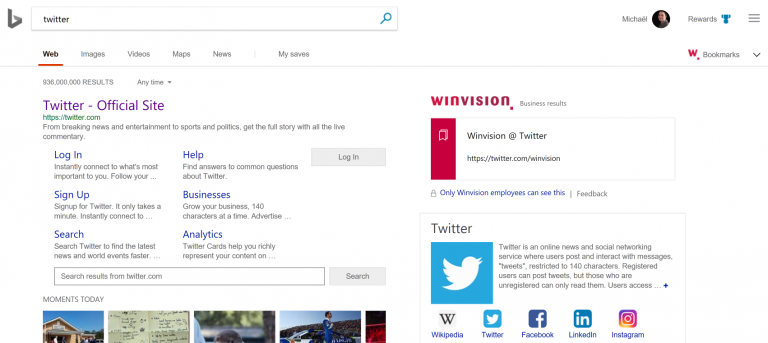**Bing - This is Twitter, my friend Glass (which is my co-rewards) ---**

The image captures the quintessential interface of Twitter, the prominent social networking service known for its concise, interactive posts called Tweets. At the top of the screen, various options are visible: web, images, videos, maps, text, websites, and the search bar. The screen also highlights the company "One Vision," with its link to twitter.com/OneVision, emphasizing that only One Vision can access this particular view. 

Below, there's a reminder that Twitter is an online platform where users can post messages limited to 140 characters. Prominent social media names like Wikipedia, Facebook, LinkedIn, and Instagram appear, illustrating the interconnected nature of modern social networks.

Further down, the screenshot includes the official Twitter site options: login, help, sign up, and business-related sections and the phrase "Let’s agree." The layout reveals a segment titled "Moments of the Day," displaying five distinct pictures, suggestive of curated highlights or trending topics. The interface is simple yet engaging, reflecting Twitter’s commitment to timely interactions and connectivity.